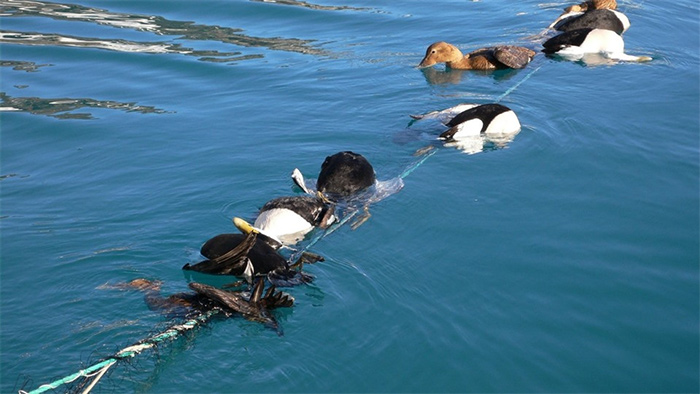The photo captures an aerial view of an ocean or river scene, revealing a distressing situation where several birds, primarily ducks but also potentially seagulls, are entangled in fishing lines or crab pot ropes. The image is taken from above, showcasing the water below with scattered land masses visible in the background. Among the birds, some appear to be alive, with one duck visibly drinking from the water while others seem to be either dead or struggling, with their bodies partly submerged. The birds show a variety of colors, including white, black, and gray, and there are about six to eight birds entangled, with two clearly deceased. Strands of plastic, presumably from the fishing gear, are also visible towards the left side of the image, adding to the overall tragic and graphic nature of the scene.